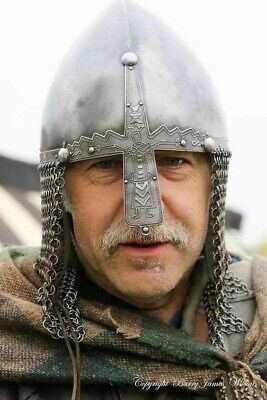This close-up color photograph captures an older man in a medieval costume, featuring a serious expression, blue eyes, and a grey mustache. He wears a silver, rustic, metal helmet with a distinct design: a rectangular nose guard extends down from the center of the helmet to the top of his upper lip, flanked by silver grommets. Surrounding his face and draping down to his neck is a silver mesh chainmail. The man is dressed in a brown and green patterned top, complemented by a rough-edged burlap scarf wrapped around his shoulders. The background of the image is a blurred white sky, emphasizing the detailed medieval attire and somber expression of the subject. The photograph is marked with the photographer's copyright.